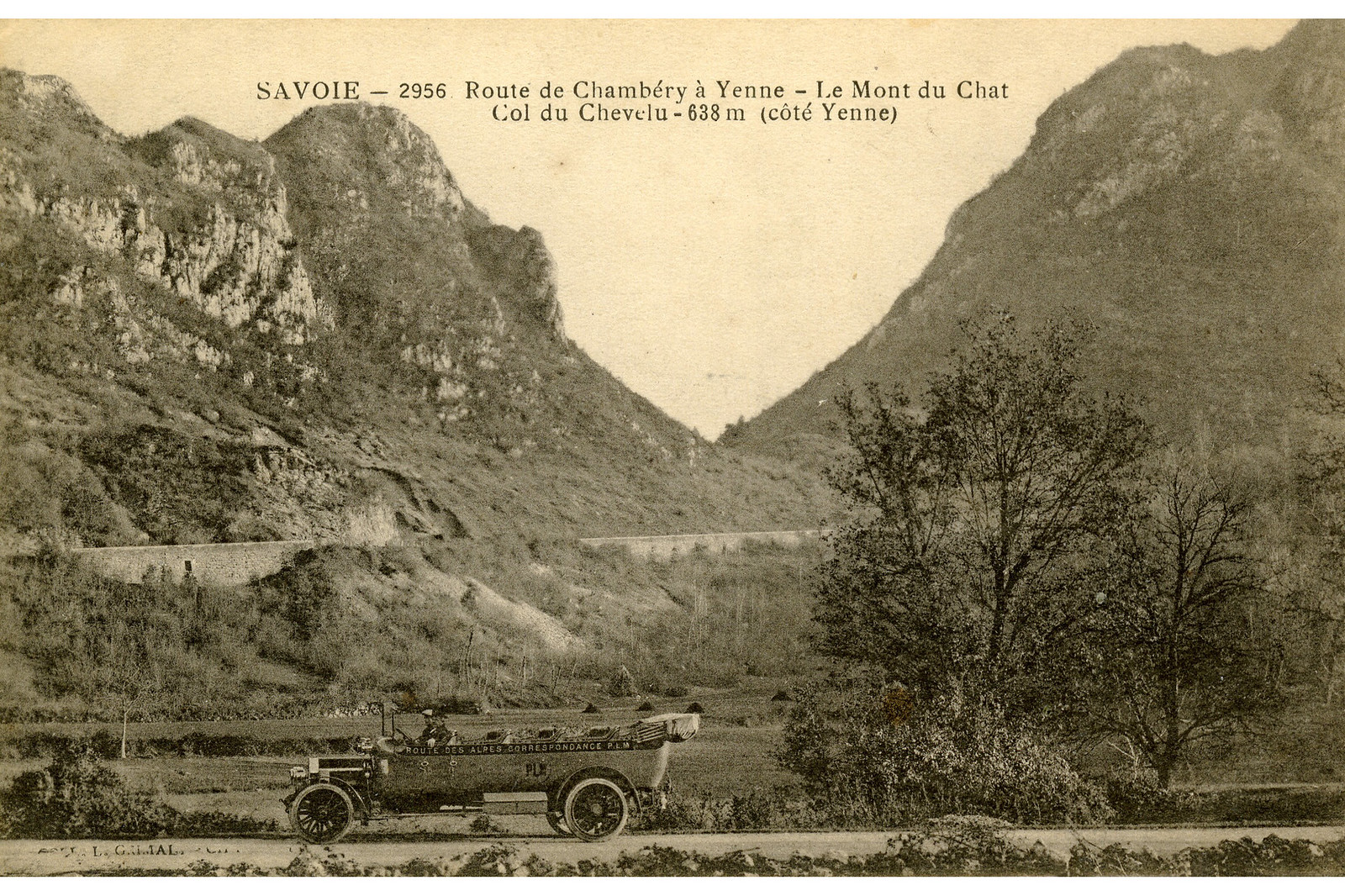This rectangular, vintage postcard, aged to a yellowed sepia tone, captures an expansive outdoor scenery. Dominating the background are large, shrubbery-covered mountains, identified by the black text over the cream-colored sky as "Savoie 2956, Route de Chambéry à Yenne, Le Mont du Chat, Col du Chablis, 638M (Côte Yenne)." Below the towering mountains lies a valley and a prominent stone wall. In the foreground, an old-fashioned, roofless car with large wooden wheels is either parked or driving along a primitive dirt road. The car, which is a six-seater, holds two visible passengers. To the right, towering trees frame the wild, undeveloped landscape, evoking a sense of timeless wilderness.